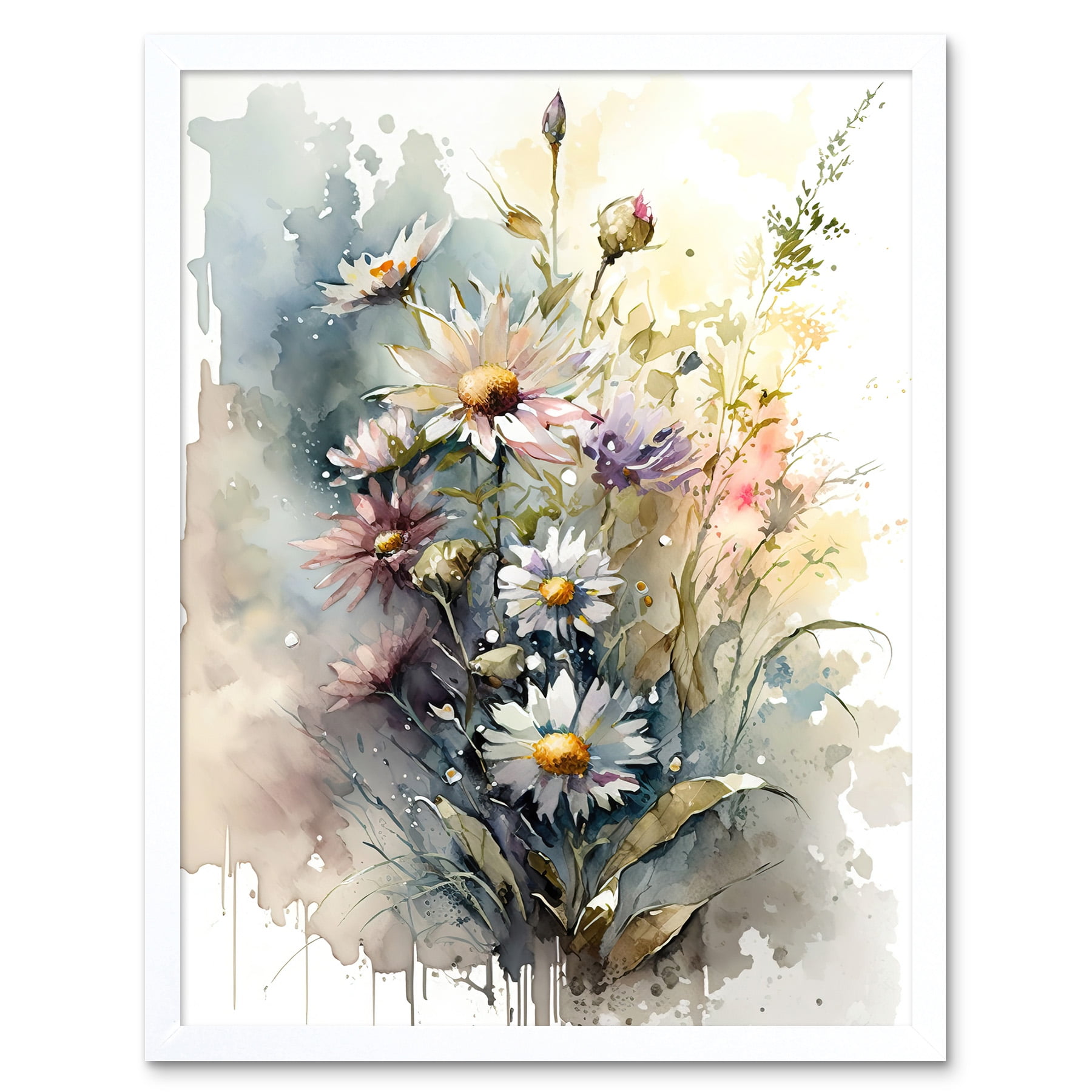This image features a painting framed with a white border, displayed against a solid white background. The painting itself has a predominantly white background with faint splashes and splotches of blue, peach, pink, yellow, and purplish-red, creating a subtle, faded effect. The central focus is a vibrant cluster of flowers, primarily resembling daisies with their distinctive, slightly jagged petals. The flowers are varied in color, including white, light pink, darker pink, purple, and magenta, with yellow centers adding a touch of brightness. Among them, some appear to be budding roses. The flowers are supported by thin and thick green leaves and tall stems, some of which seem to drip downwards, blending into the background's delicate wash of colors. The overall effect is one of a gentle, painterly scene with an impressionistic feel.